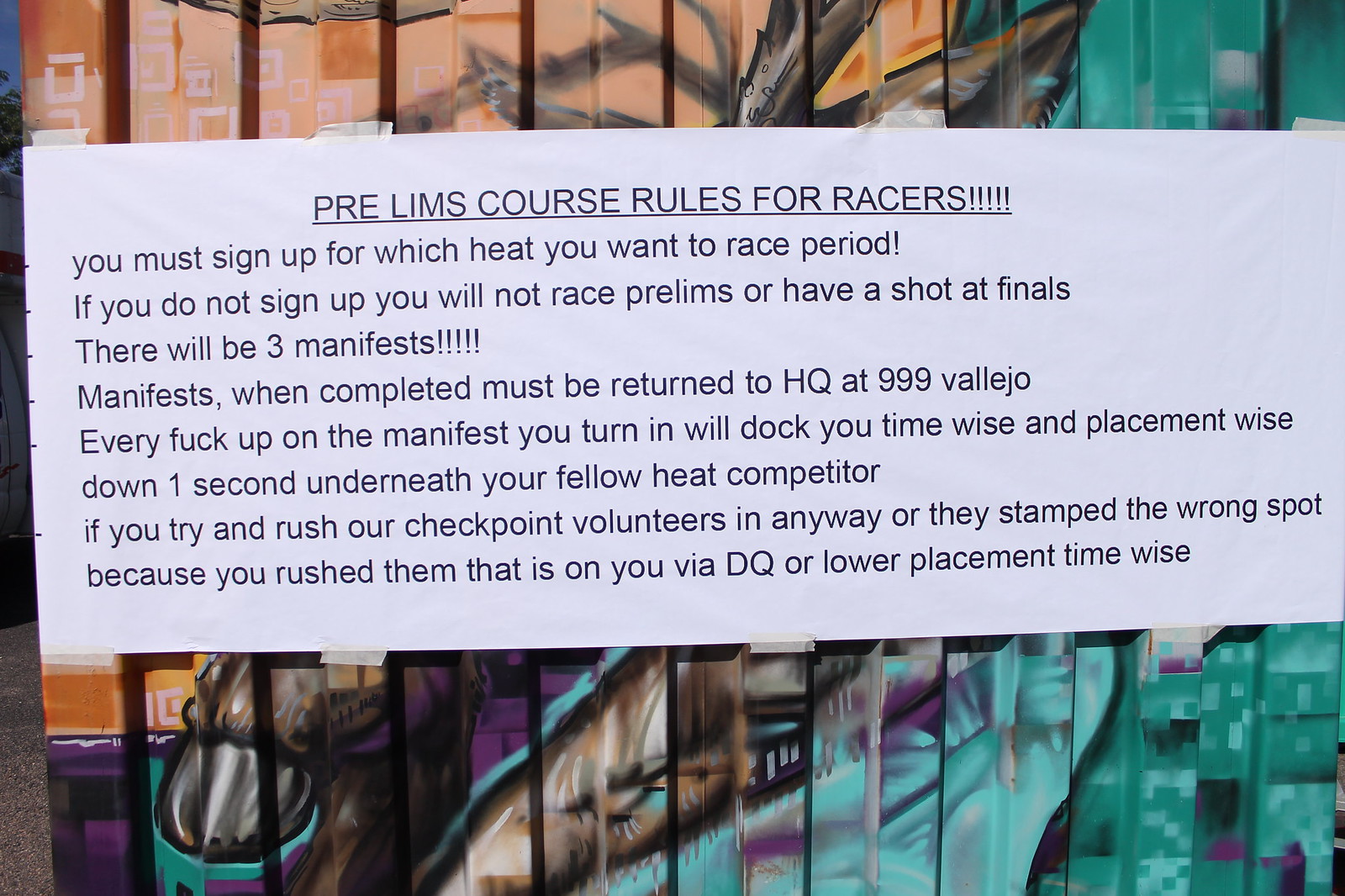The image displays a white piece of paper with black text over a light purple background, which features an indistinguishable picture with various colors, including turquoise, silver, and brown, intersected by black lines resembling a picket fence. The text titled "Prelims Course Rules for Racers" outlines the necessary guidelines for participants:
- Racers must sign up for their preferred heat to be eligible for both prelims and finals.
- There will be three manifests that need to be completed and returned to HQ at 999 Vallejo.
- Errors on your manifest will result in time and placement penalties, positioning you one second behind your heat competitors.
- Attempting to rush checkpoint volunteers, causing errors such as a misplaced stamp, will also result in disqualification or a lower placement.